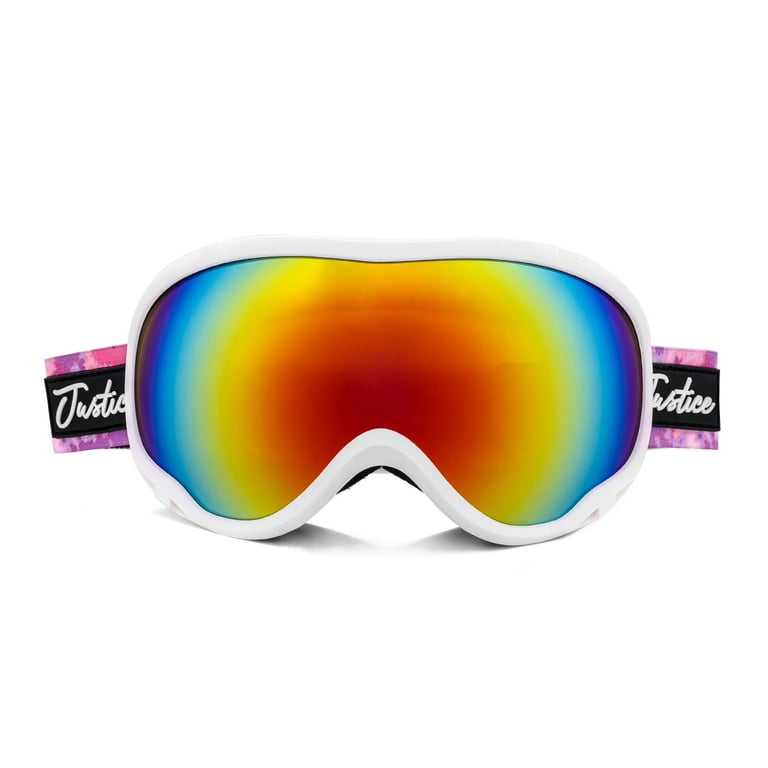The image features a pair of large snow goggles prominently placed on a white surface, casting a shadow below them. These goggles boast a reflective, multi-colored façade starting with a bright orange center that expands outward into yellow, light blue, and then darker blue, before finally transitioning into purple at the outer edges. Surrounding the lens is a white trim, and there are black accents around the very edges and the nose area. The goggles are equipped with a strap designed in a pink camouflage or tie-dye pattern with sections displaying the word "Justice" in white lettering on a black label on each side. The goggles appear to have a sturdy build and are likely intended for snowy conditions.